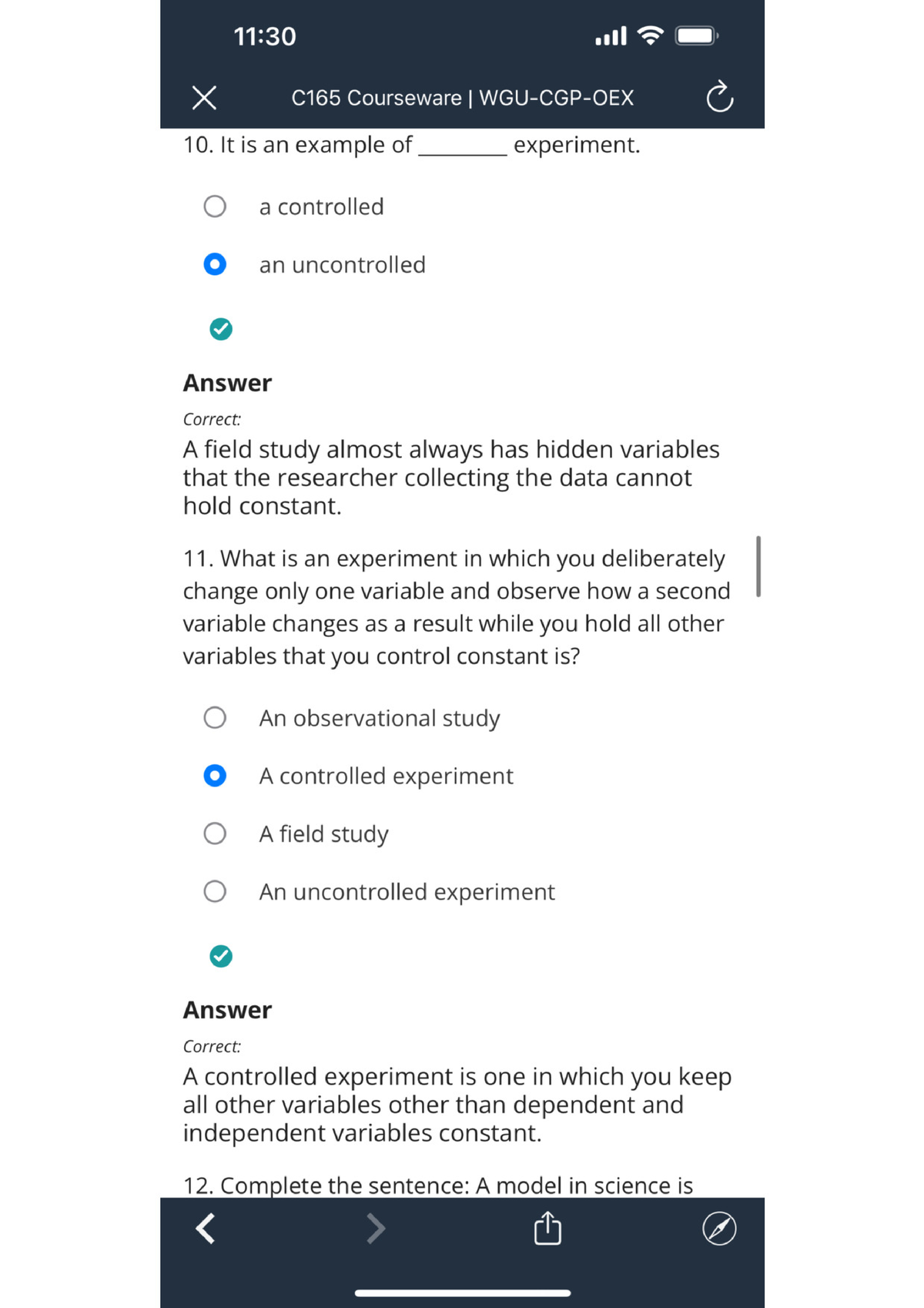This image appears to be a screenshot from a C165 courseware module by WGU tagged as "WGU-CGP-OEX," viewed likely on a mobile device. The content of the image includes multiple-choice questions primarily focusing on types of experiments. The user is engaged in what seems to be a quiz, as evidenced by marked answers and feedback.

One question presented is: "This is an example of a blank experiment," with the options being "controlled" or "uncontrolled." The user has selected "uncontrolled," which is indicated as correct with a check mark and the accompanying feedback: "Answer correct. A field study almost always has hidden variables that the researcher collecting the data cannot hold constant."

Another question, labeled "C11," asks: "What is an experiment in which you deliberately change only one variable and observe how a second variable changes as a result while you hold all other variables that you control constant?" This question offers four choices, among which "controlled experiment" is selected and marked correct with the explanation: "Answer correct. A controlled experiment is one in which you keep all other variables other than dependent and independent variables constant."

The image cuts off just before "Question 12," revealing a black rectangle at the bottom, indicating the edge of the smartphone screen. The display shows the beginning of the next question but does not provide further details.

Overall, the image captures a moment of interactive learning, highlighting the principles of controlled and uncontrolled experiments in a structured educational setting.